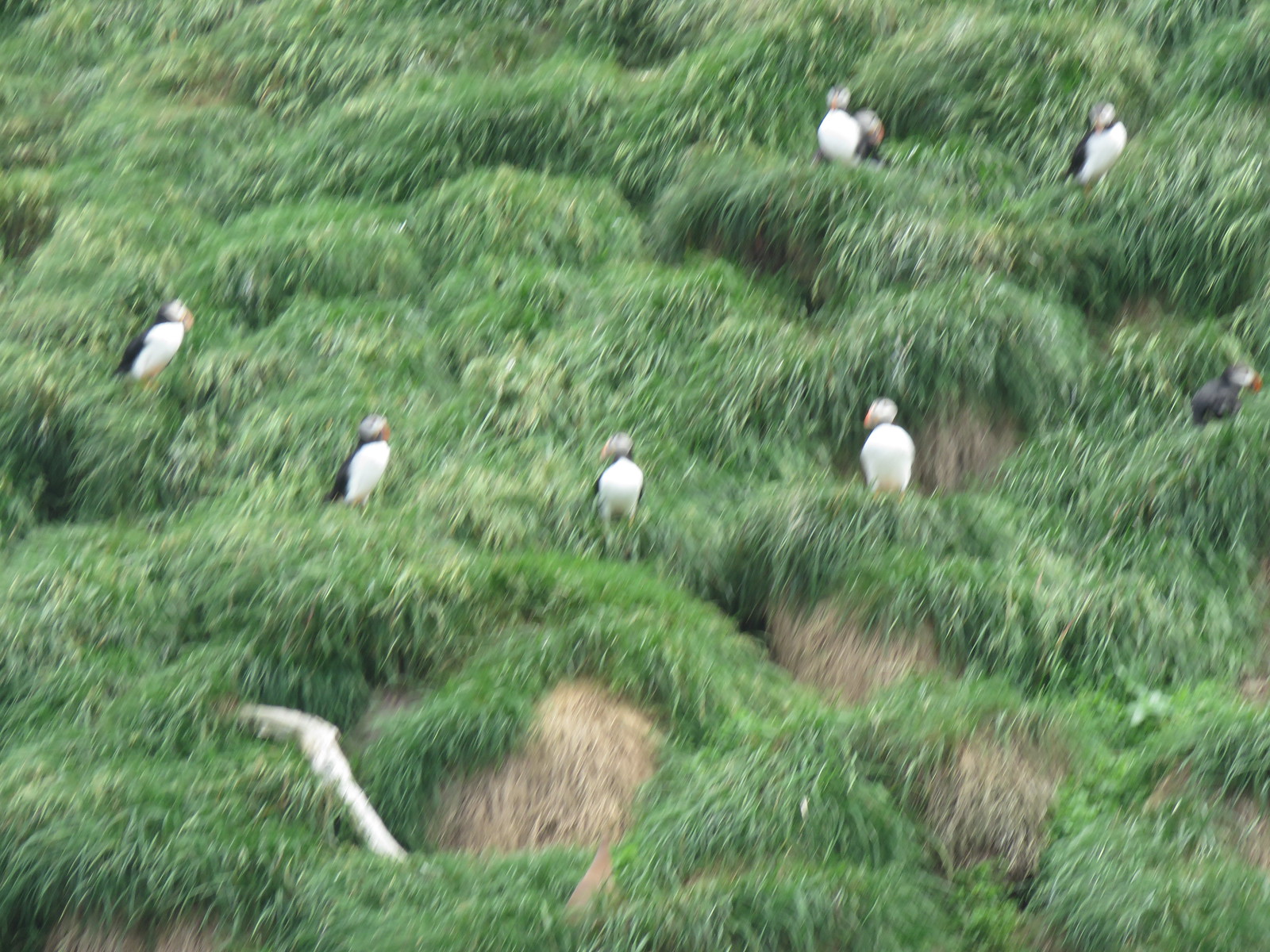This extremely zoomed-in, grainy photo taken outdoors features a hillside overgrown with long, wavy green grass interspersed with patches of dead grass. The focus, though blurry, is on a group of five birds arranged in a U-shaped formation on the hill. Resembling penguins or small toucans, these birds have distinctive white bellies, black backs, and short orange beaks. One bird, positioned at the far right, clearly shows its black back. Scattered evenly apart, they stand amidst the lush greenery, with an area of exposed hay-like ground in the middle. Towards the bottom left of the image lies a fallen, pale tree log, adding to the natural setting. Although the image lacks clarity, the contrasting colors of the birds and the verdant backdrop create a vivid impression of a serene, hillside scene teeming with wildlife.